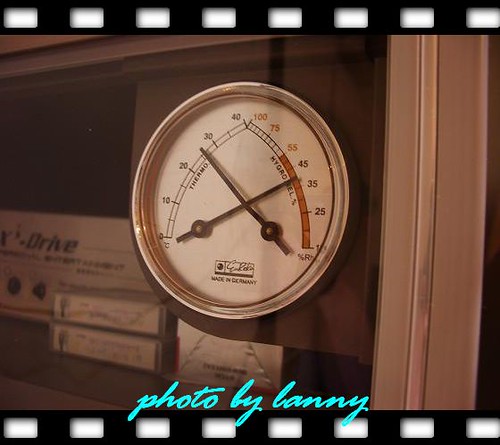This image features a close-up of a round analog thermometer with a black circular frame, reminiscent of an old-fashioned watch. The thermometer is mounted on a glass window, providing a glimpse of objects resting on a table or within a shelf behind it. The photograph is bordered on the top and bottom by a design that looks similar to the sprocket holes of a film strip, with evenly spaced white rectangles on a black background.

The face of the thermometer displays numerical markings in increments of 10, ranging from 0 to 100, with two hands pointing to specific values, likely indicating the current temperature. A red line enhances the clarity of the reading. A teardrop-shaped emblem, also annotated with the numbered scale, suggests a design focused on precision.

The caption "Photo by Lanny" is inscribed at the bottom, attributing the work to the photographer. The image combines an element of nostalgia with a practical device, capturing the essence of temperature measurement in an aesthetically appealing frame.